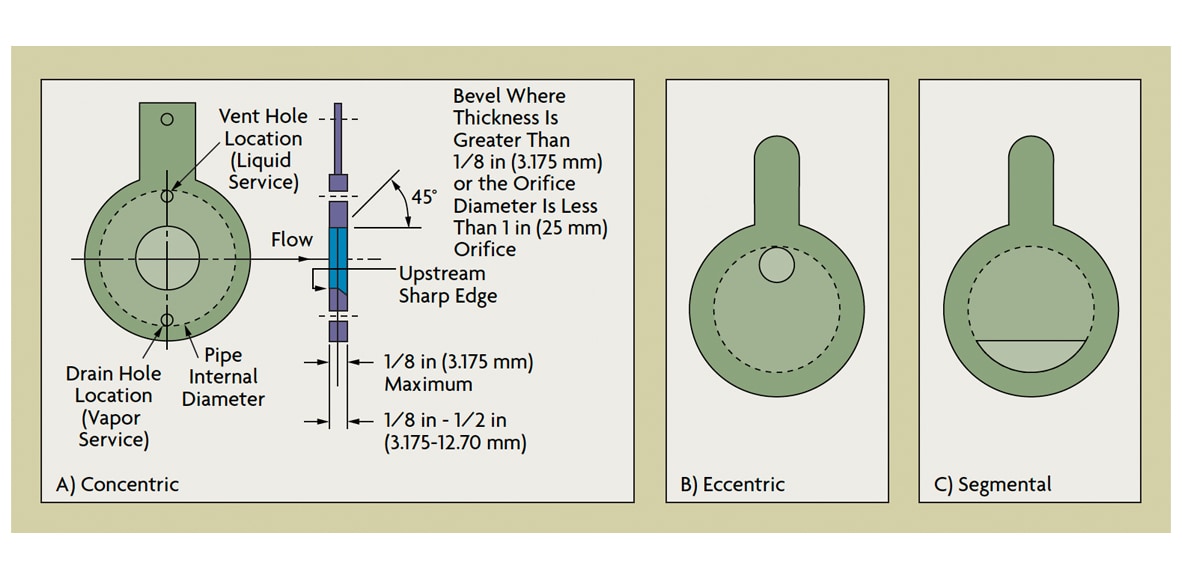The image is a detailed scientific diagram of a piping mechanism, split into three sections labeled A, B, and C, showcasing concentric, eccentric, and segmental views respectively. Each section depicts a green pipe with different internal angles and measurements associated with liquid and vapor services. 

At the top, there is a vent hole location labeled for liquid service, while a drain hole is marked for vapor service at the bottom. The diagram includes information regarding pipe internal diameter and various specifications for flow, including a hand-drawn area in blue and purple showing upstream flow, a sharp edge of a maximum one-eighth inch, and beveling details where applicable.

The textual information is primarily in black, indicating critical annotations such as "1/8 inch to 1/2 inch bevel where thickness is greater than 1/8 inch or the orifice diameter is less than one inch." Each diagram section is framed in light tan against a white background, adding clarity to the delineations. This schematic is designed to provide a precise representation of the piping mechanism through its detailed views and annotations.